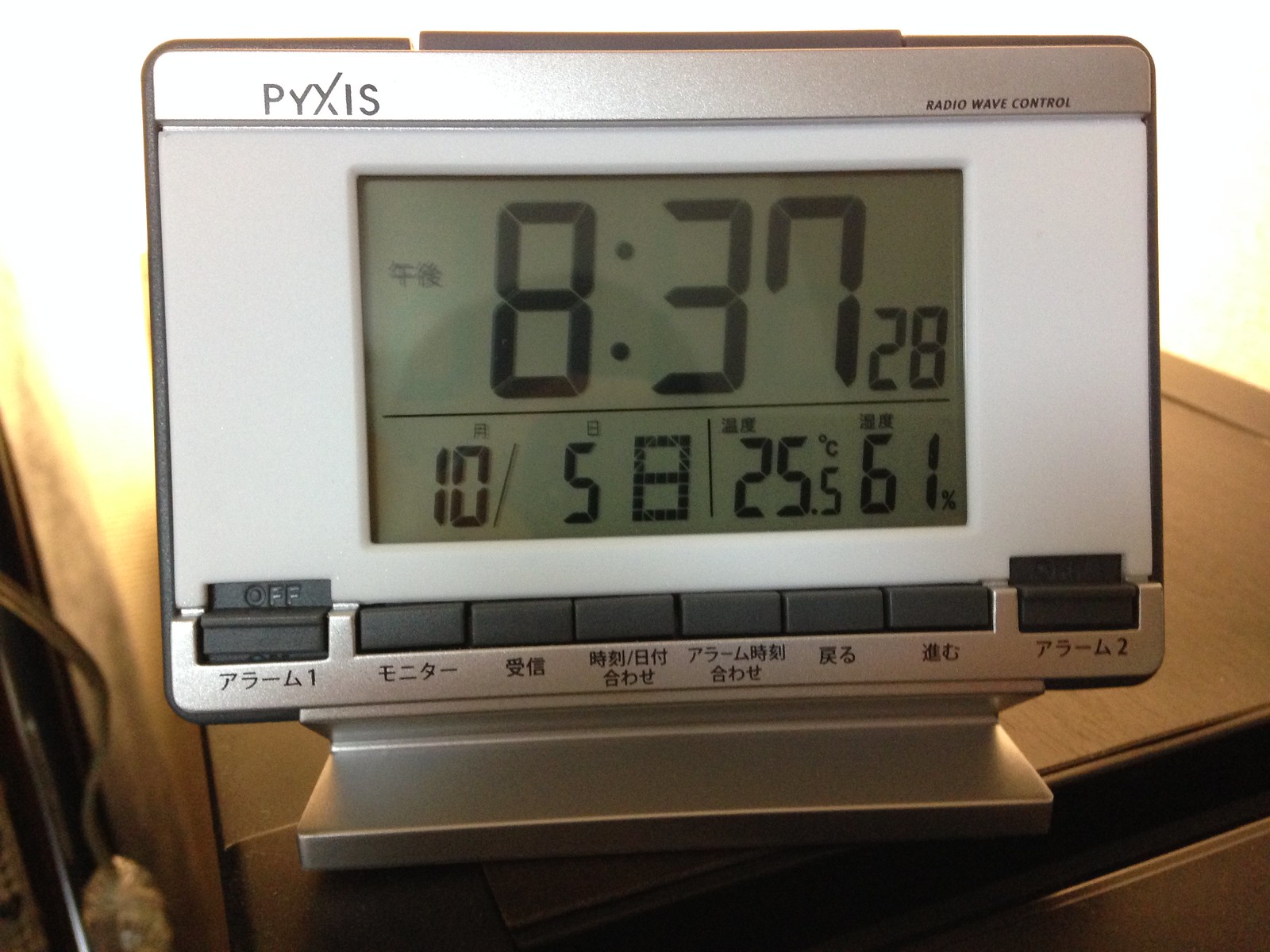This rectangular landscape-oriented photograph captures a close-up shot of a sleek, silver-toned digital clock with integrated thermometer and LED display, positioned upright on a woodgrain end table. The clock's face features a white background with a typical greenish LCD screen displaying the time 8:37:28. The temperature reading below shows 25.5 degrees Celsius. The other indicators on the clock are inscribed in an unidentified Asian script. At the top of the clock, a silver panel is adorned with the text "Radio Wave Control." A light source, likely a lamp, illuminates the scene from behind, casting a subtle glow, while a curtain is partially visible to the left, adding to the cozy interior ambiance.